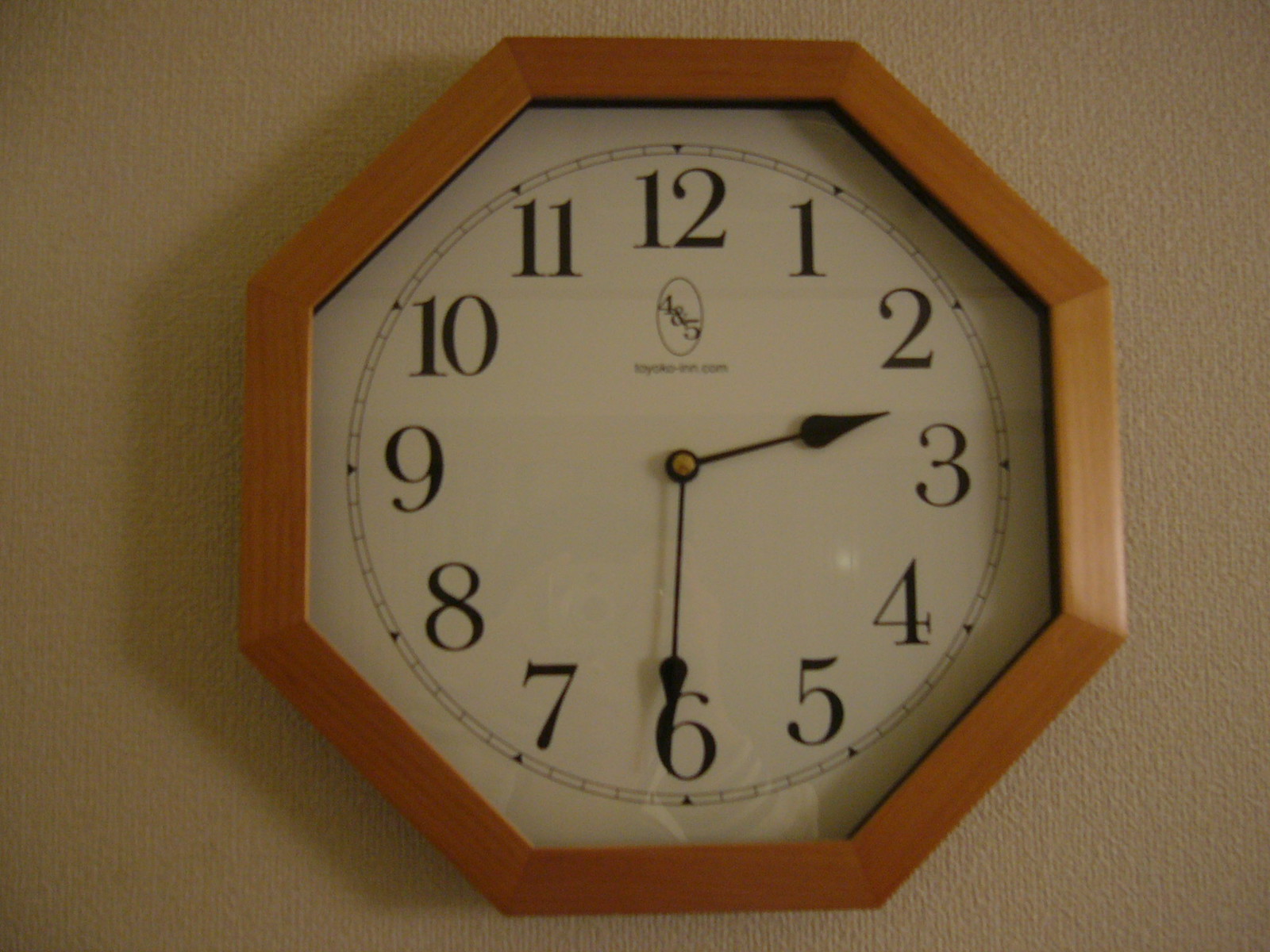This image captures an octagonal clock hanging on a dark beige wall. The clock's frame is a medium brown wood grain, imparting a classic and elegant look. The time displayed is precisely 2:31. The clock face is white or off-white, providing a clear contrast to the large, bold black numbers that mark each hour from 12 to 11. Notably, there are no second hands on this clock, just the hour and minute hands, which are also black with a gold center, enabling easy readability. In the middle of the clock face, there is a reflective oval shape where the numbers '4' and '5' are printed, and beneath it, additional black writing which is not entirely legible. Surrounding the numerals are smaller increments between each hour, indicated by fine lines. The entire setup reflects a slightly dim photographic condition, with a reflective surface in the clock hinting at the presence of the photographer.